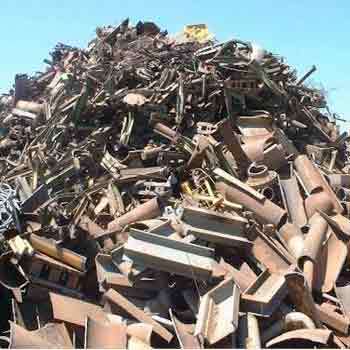A massive landfill spreads across the image, dominated by an enormous mountain of diverse construction debris and metal scrap, occupying nearly 90% of the frame. The jumble of discarded materials forms an arc that reaches up towards a cloudless blue sky, which is only visible in small portions at the top corners of the image. The pile consists of a chaotic array of items, including rusted brown and silvery metal fragments, yellowish pieces, ceramic pipes or roof tiles, and steel I-beams. Among the debris are various shapes and sizes of discarded objects like I-beams, pots, building materials, and containers. Some metal pieces stick out dangerously from the pile. A brush of vegetation can be seen towards the top of the heap, adding to its chaotic appearance. This scene of disorder illustrates what appears to be a junkyard or disposal area, hinting at the potential hazards of navigating through such treacherous terrain cluttered with sharp and uneven debris.